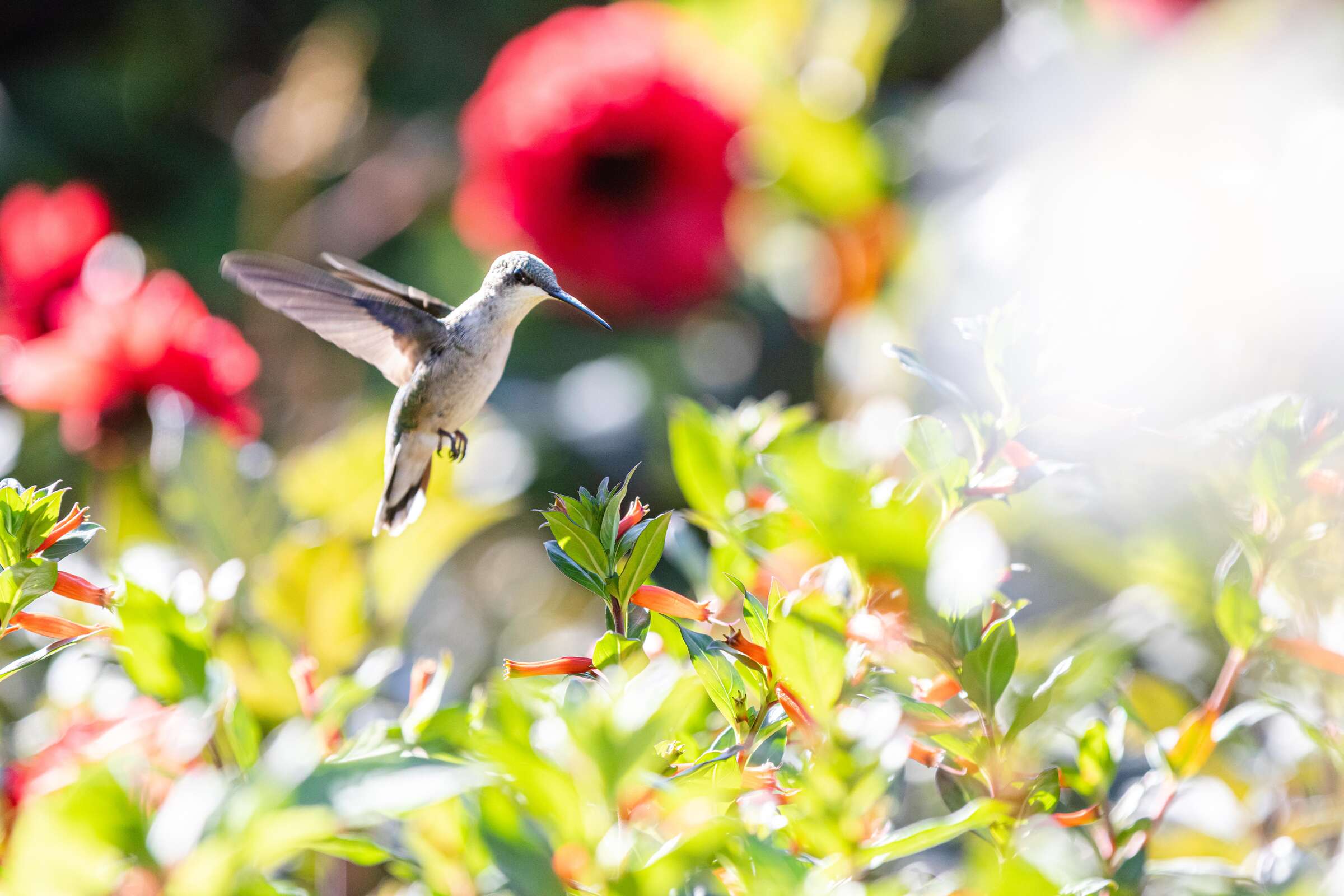This vibrant color photograph, taken outdoors during the day, captures a close-up of a hummingbird in mid-flight, seemingly hovering with grace. The hummingbird, with a grayish-black body and a light, cream-colored underbelly, exhibits intricate details; its black beak points forward while its wings are outstretched and curved backward. The bird’s tiny feet are curled up in front of its body, indicating a poised position as if preparing to land. It is feeding on the trumpet-shaped, red bell flowers of a lush vine shrub. Behind it, the background showcases more of these red flowers and leaves, although the foliage and some flowers are out of focus, enhancing the emphasis on the bird. A significant sunbeam enters from the top right, causing a lens flare that slightly whites out part of the photograph, adding to the dreamy and sunlit atmosphere. The fine details and lighting bring a sharp focus to the hummingbird, making it the undeniable focal point of this elegant and dynamic image.